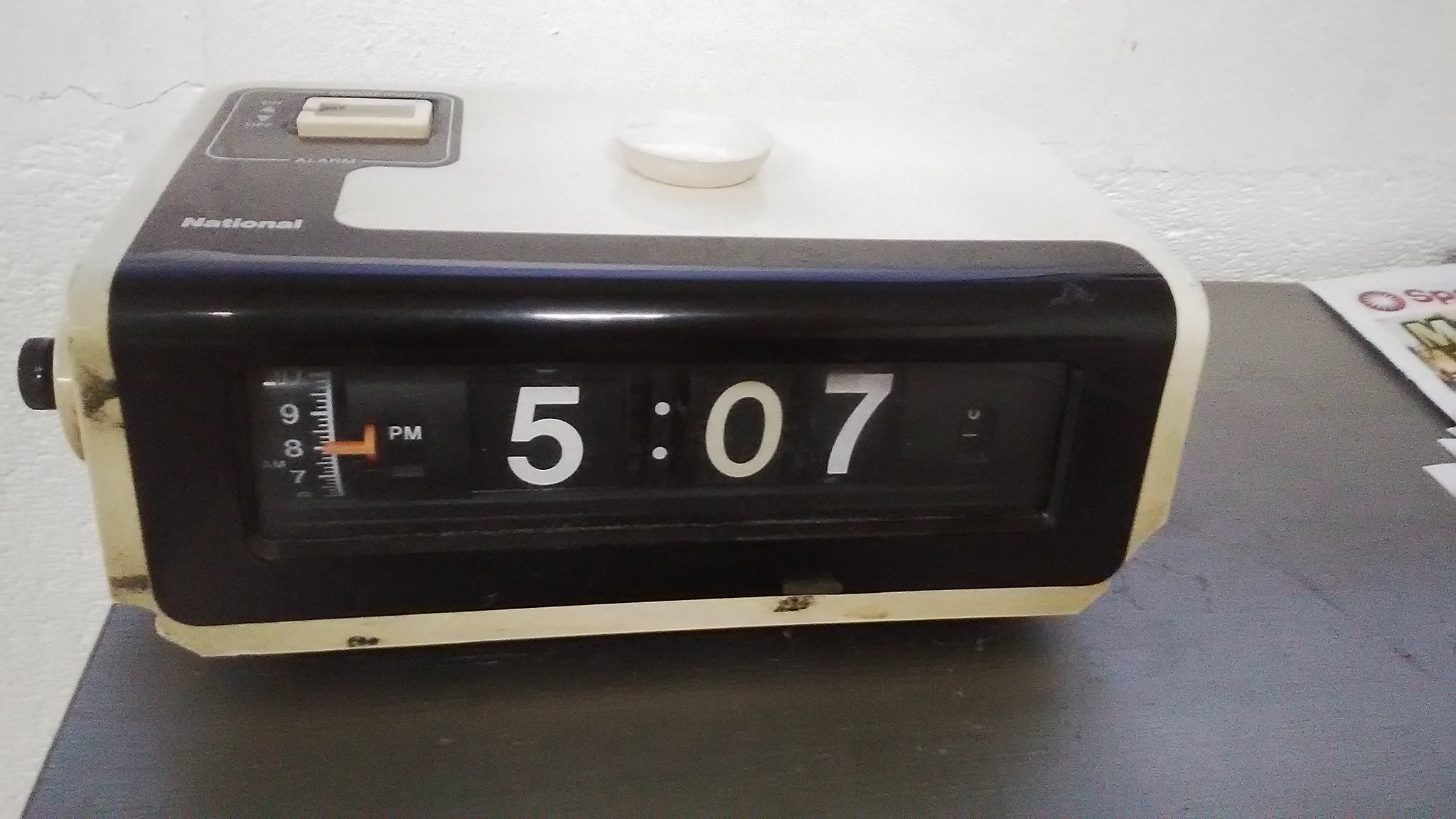The image features a vintage-style plastic alarm clock branded "National," prominently displayed with a black front and a contrasting white frame and top. The clock face includes a rotating dial mechanism used to set the time. The digital display currently reads 5:07 PM. The device is slightly elevated, supported by small feet or a beveled edge. Additionally, there is an intriguing gauge with a red arrow pointing to the number 8, the function of which is unclear but may relate to the alarm settings. The clock is positioned on a grey table, with a few scattered papers visible in the top right corner of the frame.